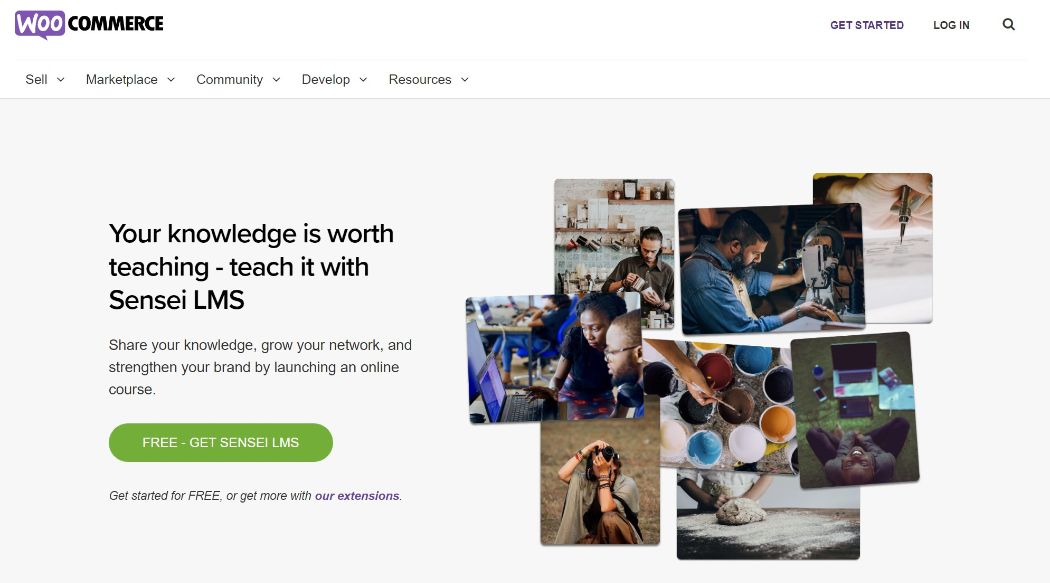Screenshot of the WooCommerce website displayed. The logo features the word "Woo" in white text within a purple speech bubble. At the top, navigation options include "Get Started," "Log In," and a search function. Below this, a horizontal menu bar lists categories: "Sell," "Marketplace," "Community," "Develop," and "Resources," each with their own drop-down menus.

The main advertisement promotes Sensei LMS, an online course platform. The highlighted text reads, "Your knowledge is worth teaching, teach it with Sensei LMS." It suggests that users can "Share your knowledge, grow your network, and strengthen your brand by launching an online course." Imagery depicts a diverse group of individuals teaching various subjects such as paint mixing, photography, cooking, sketching, and computer skills.

A prominent green button offers, "Get Sensei LMS for Free" with an option to "Get More with Our Extensions." The advertisement suggests that the platform is reminiscent of educational sites like CuriosityStream, but focuses more on instructional content delivery.